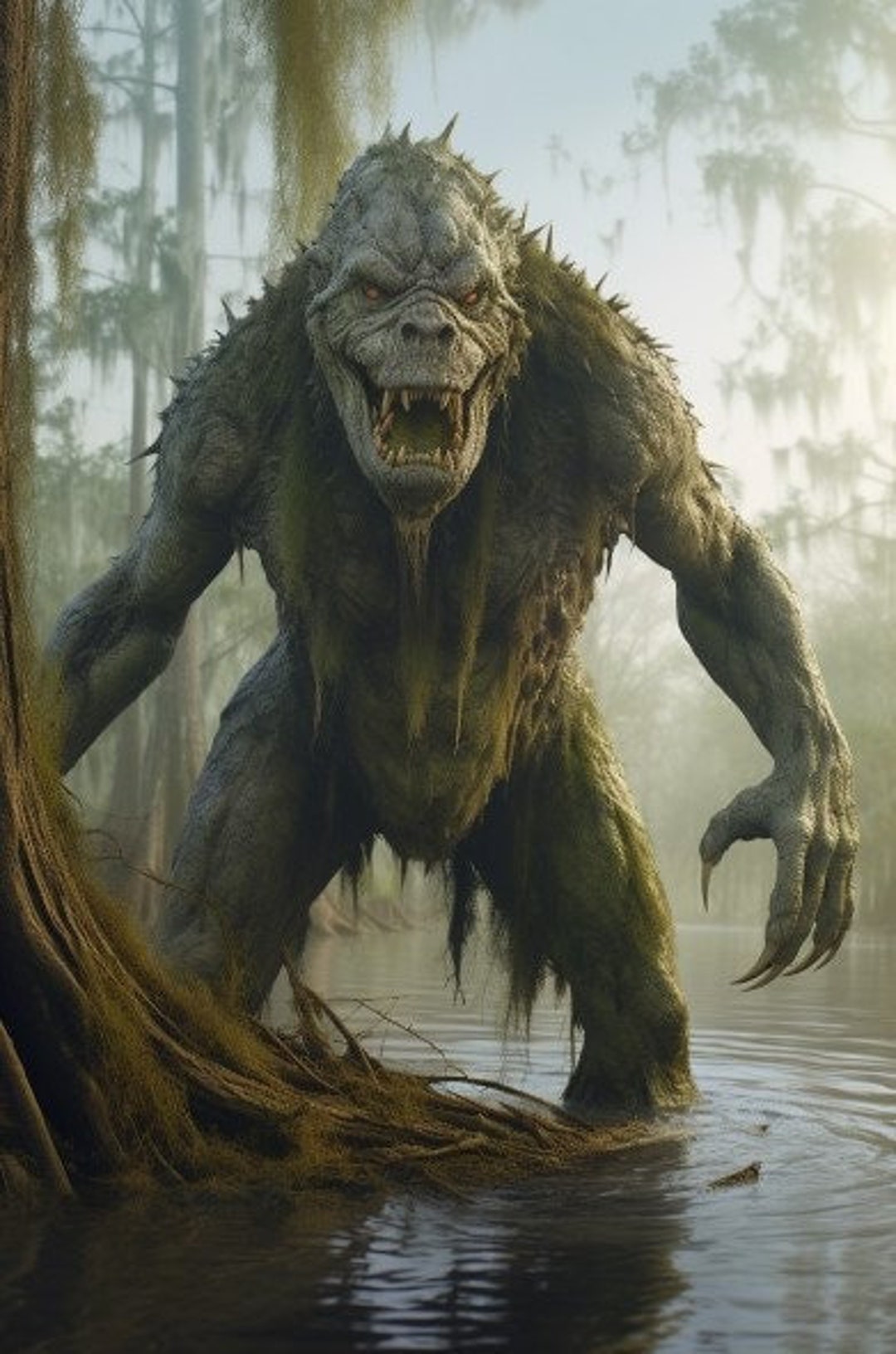This detailed image appears to be a still from a movie or a graphic poster featuring a monstrous creature in an eerie outdoor setting. The green-skinned, gorilla-like monster stands menacingly in murky, dark water with a jungle backdrop featuring trees draped in Spanish moss and the silhouettes of vegetation and tree trunks around him. The creature's physique is imposing, characterized by a tall, muscular build with broad, rounded, and hunched shoulders, thick thighs, a narrow waist, and long, muscular arms with sharp, clawed fingers. It has a fur-covered chest and legs, with hair sprouting in tufts around its shoulders and head. The monster's facial features resemble a grotesque hybrid of a gorilla and a dinosaur, with a long, gnarly face, a nose like that of a gorilla, and a mouth agape to reveal yellowed, sharp fangs. Its eyes are wide open in a fierce growl. The overall scene has an eerie, fuzzy cast, possibly illuminated by the light of dawn or dusk, casting a surreal quality to the surroundings. The sky behind the creature is a pale blue with faint sunlight filtering through the trees, enhancing the dark, enigmatic atmosphere of this swampy jungle.